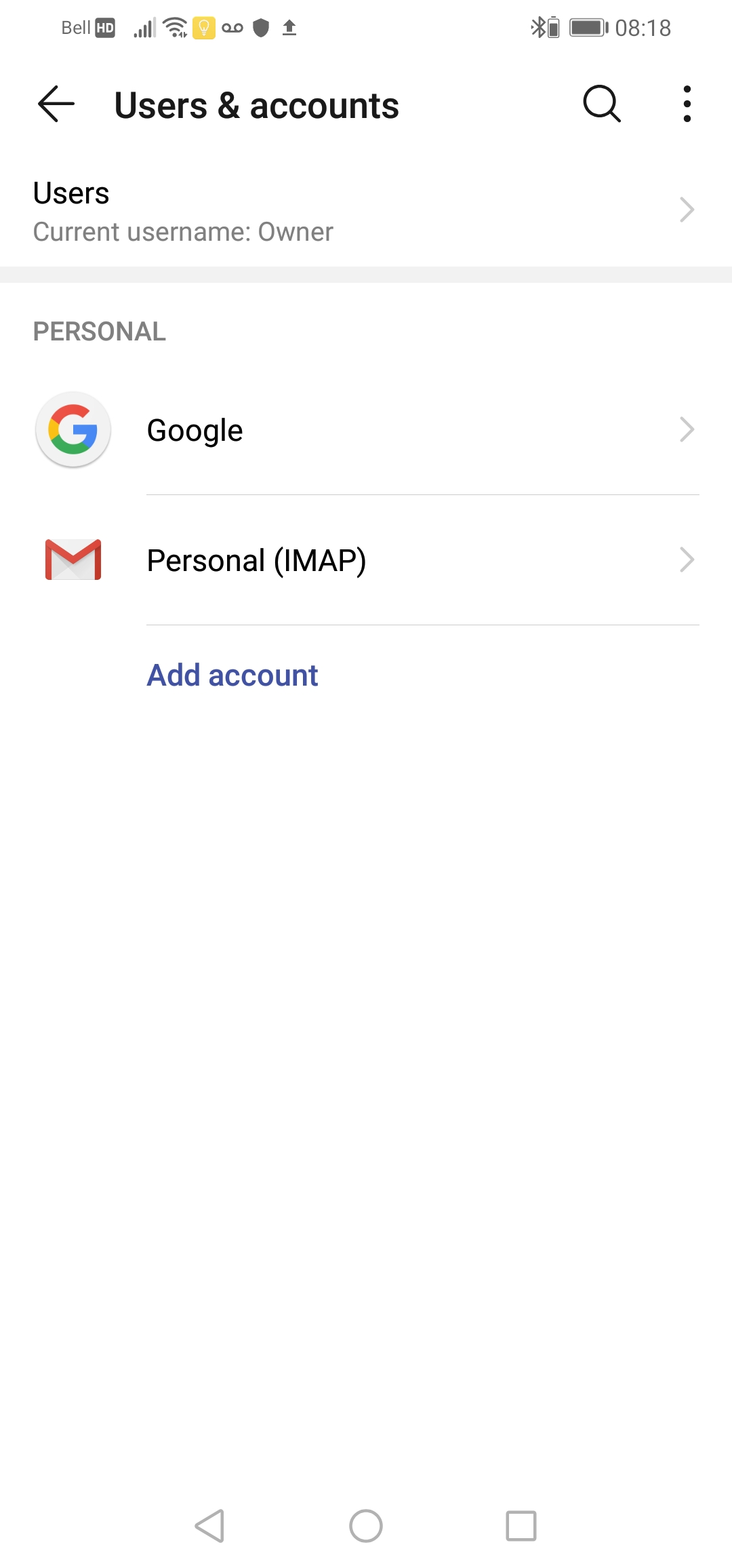The image captures a smartphone screen displaying the "Users and Accounts" section of a Google account, inclusive of Gmail. The timestamp at the top of the screen shows 8:18, and the battery icon indicates it is almost fully charged. The status bar also includes a Bluetooth symbol and a few unclear notification icons. An arrow pointing left and a search icon, accompanied by three vertical dots, are visible, indicating navigation options and additional settings.

Within the main content, the section labeled "Users" displays the "Current Username" under "Owner" in the "Personal" account category. Below this, the Google icon is prominently featured next to the word "Google." Directly beneath it is the Gmail icon, labeled "Personal, IMAP," denoting the signed-in email account type. A blue "Add Account" option is visible at the bottom, inviting the user to incorporate another account. Despite the presence of subtle notification icons, their specific details remain indistinguishable.